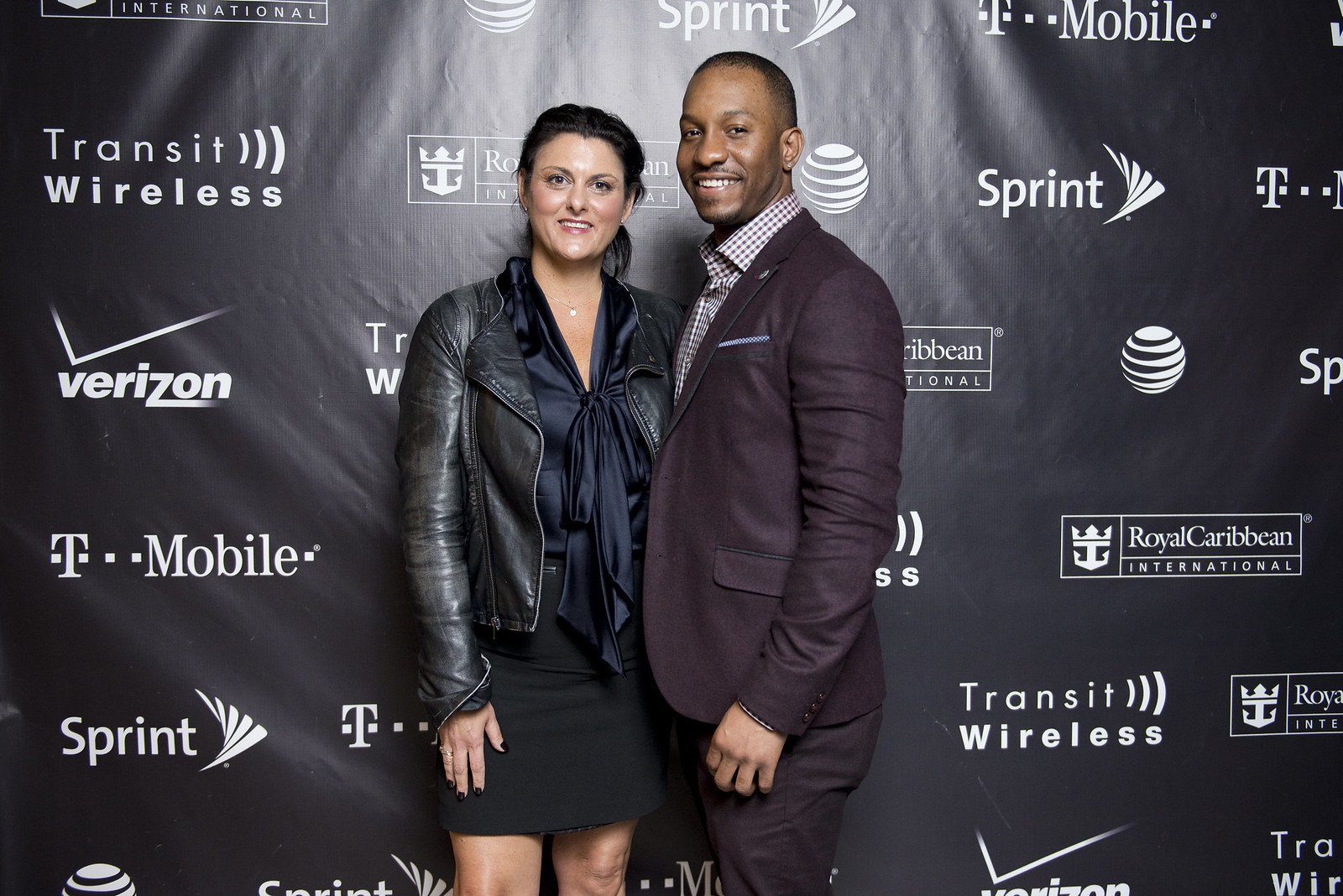In this color press photo, a well-dressed African-American man and a woman pose in front of a black press banner emblazoned with white logos of various brands, including Transit Wireless, Verizon, T-Mobile, Sprint, and Royal Caribbean International, highlighting their sponsorship of the event. The man exudes elegance in a purple or blue blazer and matching dress pants, paired with a checkered white button-up shirt. Standing next to him, the woman, potentially of Latina, Middle Eastern, or white descent, has her long black hair pulled back into a ponytail. She dons a chic outfit, consisting of a black satin blouse with a bow tie at the front, a black leather jacket, and a short black skirt. Both individuals are smiling warmly at the camera, clearly posing for the press at this sophisticated event.